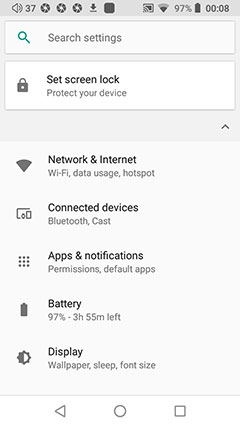This screenshot captures various details from a smartphone's settings dashboard. At the top left, the volume level is shown to be at 37%. To the right of the volume icon, there are several other icons including a Wi-Fi icon, and a battery icon indicating 97% charge. The time displayed at the top right reads 00:08.

Below this section, a white rectangle with a teal magnifying glass icon is visible, bearing the text "Search settings". Directly beneath this, there is a black lock icon accompanied by the text "Set screen lock" and "Protect your device", all enclosed within another white rectangle.

The next portion of the screenshot features a white background divided into various sections. The first section reads "Network & Internet" followed by details such as "Wi-Fi, data usage, and hotspot". Further down, there is a gap in the text, after which it reads "Connected devices" with options for "Bluetooth" and "Cast".

Another gap in the text is evident before the next section, which reads "Apps & notifications" listing "Permissions" and "Default apps". Continuing, the next line shows "Battery", repeating the 97% charge along with an estimated 3 hours and 55 minutes of battery life remaining.

Lastly, another text gap appears before the final section labeled "Display", which includes options for "Wallpaper, sleep, font size".